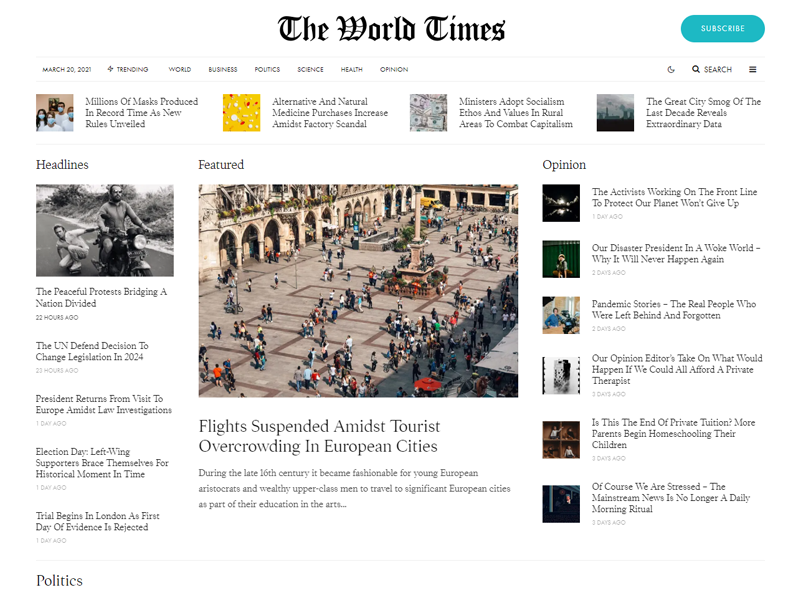In the image, we see the homepage of The World Times. The header prominently displays "The World Times" in a distinctive Medieval Times-inspired font in bold black text. On the top right corner is a blue "Subscribe" button, inviting readers to stay updated.

Just below the header, a thin horizontal line stretches across the width of the page, immediately followed by the issue date, "March 2021." Beneath the date, a navigation bar lists various menu options: "Trending," "World," "Business," "Politics," "Science," "Health," and "Opinions," allowing readers to explore different sections of the newspaper.

The main body of the page displays four articles in a row, each accompanied by a small thumbnail image. The articles are organized into rows with distinct labels. The first row is titled "Headlines," showcasing the top news stories. The second row, labeled "Featured," includes highlights such as "Flights Suspended Amidst Tourist Overcrowding in European Cities," capturing current global issues.

On the right side of the page, a third column titled "Opinion" features articles with corresponding thumbnail images. The first opinion piece, "The Activists Working on the Front Line to Protect Our Planet Won't Give Up," discusses the dedication and resilience of environmental activists.

The layout is clean and organized, ensuring readers can easily navigate and find the topics of interest.